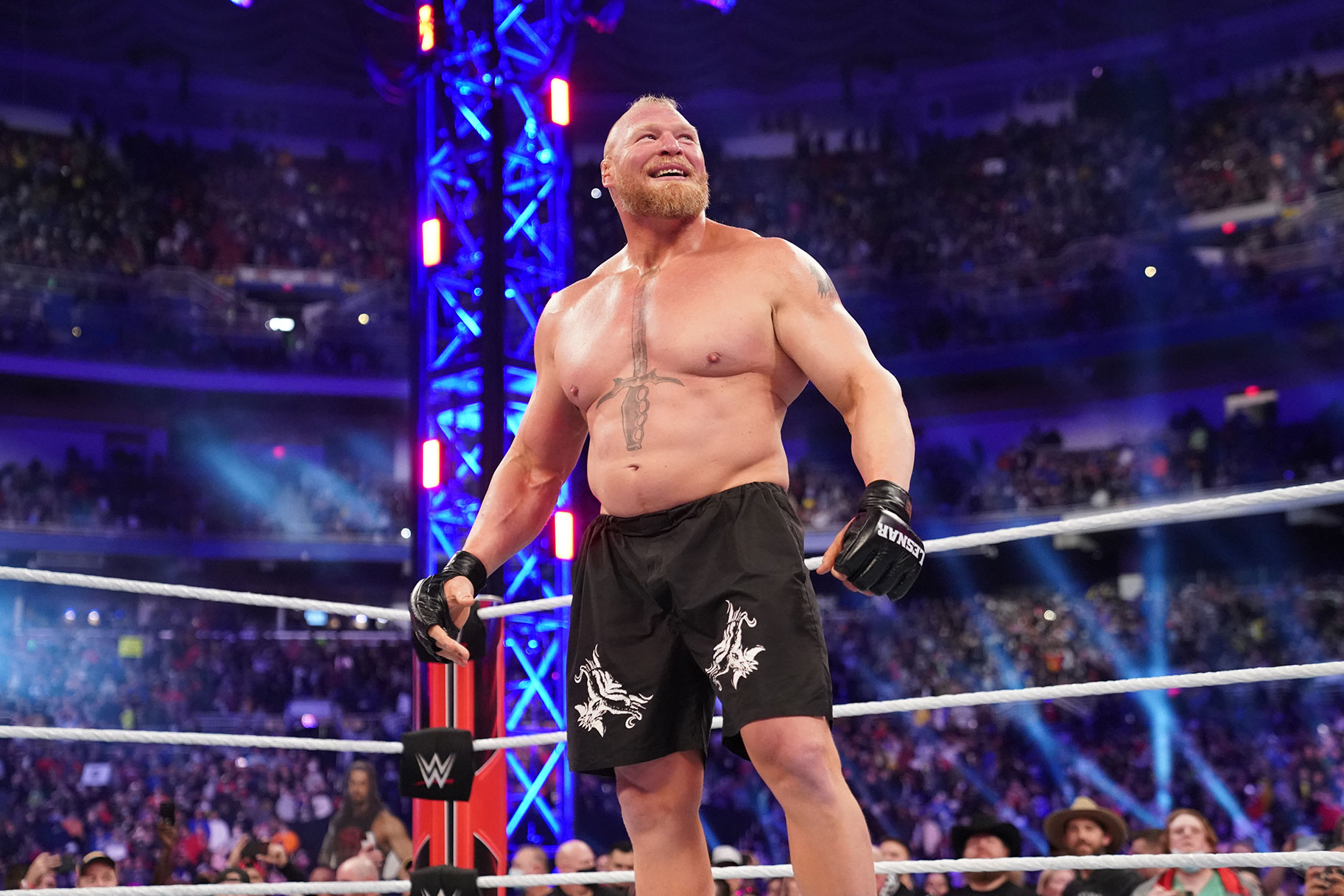In the middle of a packed, three-tiered amphitheater stadium aglow with purple and blue neon and strobe lights, professional wrestler Brock Lesnar stands confidently in a boxing ring. The darkened stadium is buzzing with a vast crowd filling every layer. Metal scaffolding, likely bearing spotlights and a scoreboard, forms a backdrop to the electrifying scene. Lesnar, with his fair skin, light blonde hair, and prominent tattoos—including a striking sword tattoo on his chest—stands center stage. He is wearing black shorts decorated with white designs, possibly featuring skulls, and black MMA gloves adorned with white lettering. His fighting stance shows his left leg slightly forward, arms at his side. He looks up and to the left with a characteristic smirk, capturing the attention of the audience.